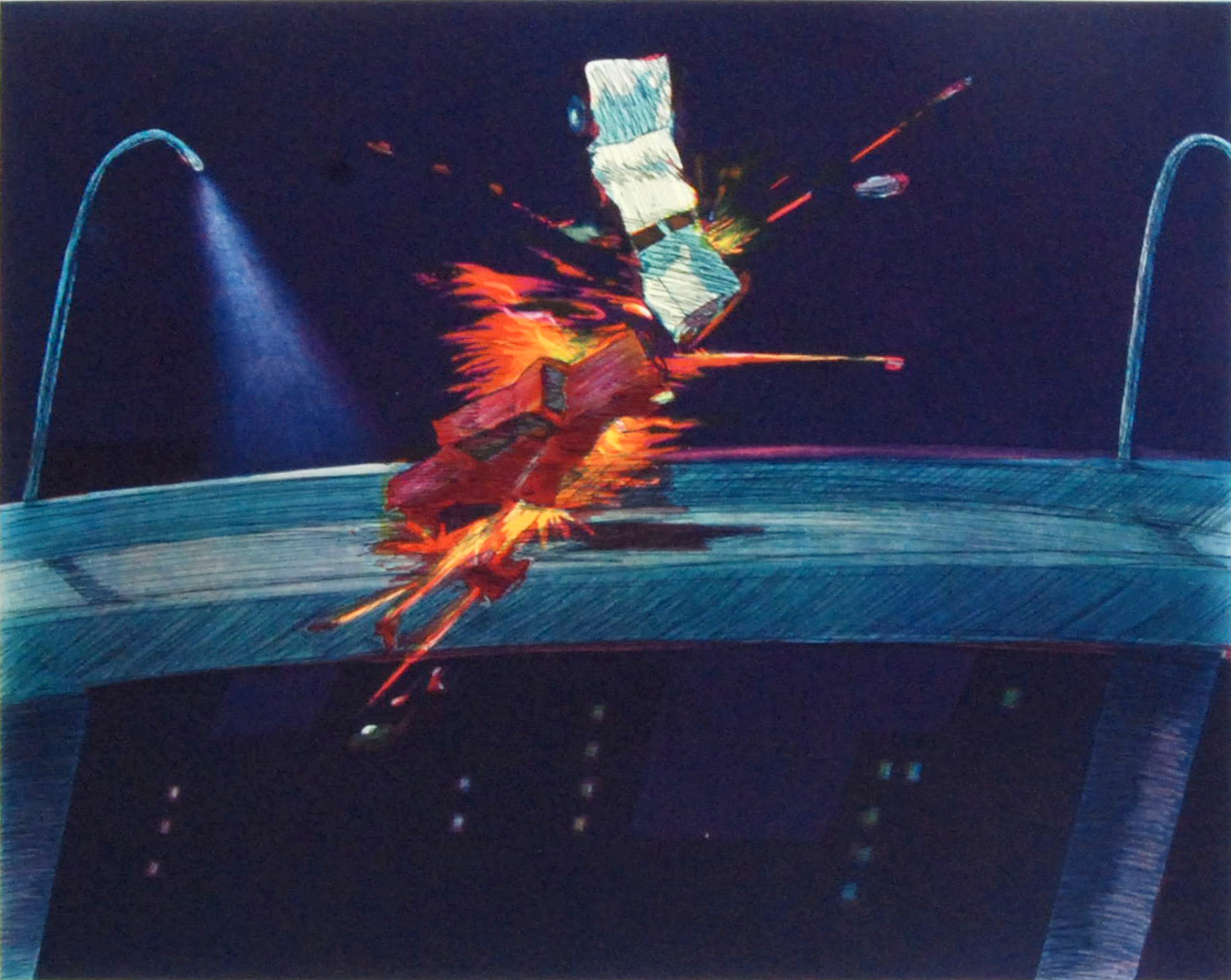This dynamic and visually striking painting vividly depicts a catastrophic car crash occurring on a high city bridge at night. Rendered in what appears to be acrylic with hints of pencil, the night sky above is a deep, dark purple, transitioning into a dark blue-black hue. The background features the silhouetted shapes of skyscrapers, their windows aglow with yellow light, creating an illuminated cityscape below the bridge.

Two cars, a red and a white one, are the focal point of the scene. The red car is engulfed in fierce flames of yellow, orange, and red, dramatically elevated on its back wheels and angled toward the top right corner of the painting. The white car, appearing grayish-blue in color, is completely airborne, flipping skyward in a chaotic arc, contributing to the sense of motion and intensity. The collision scene is depicted with detailed explosions of fire and fragments of car parts scattering in all directions.

Adding to the drama, two street lamps are featured, with one prominently casting light on the bridge’s surface and illuminating the fiery wreckage. The combination of the dark, atmospheric night sky, the fiery explosion, and the stark illumination from the streetlights creates a high-contrast, almost surreal cartoon-like aesthetic, capturing the sheer energy and chaos of the collision.